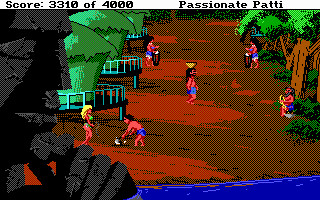This colorful screenshot from a retro video game, possibly named or featuring a character called "Passionate Patty," shows a vibrant tropical island setting. At the top of the screen, the score reads "3310 of 4000" in small black font. Dominating the scene is a blonde-haired woman in green, who stands out as she walks towards a man near one of three green huts perched on posts with metal railings around their decks. Several characters with red-orange skin and black hair, dressed in blue shorts, are scattered around the island; some are standing, talking, working, or carrying a basket on their heads. The ground is a distinct red-brown dirt, with patches of black rocks and green leafy trees adding to the lush environment. A small creek or shoreline of a river is visible in the bottom right corner. Prominently in the foreground to the left, there is a stone statue of a man's face resting his hand under his chin, exuding a pensive demeanor.